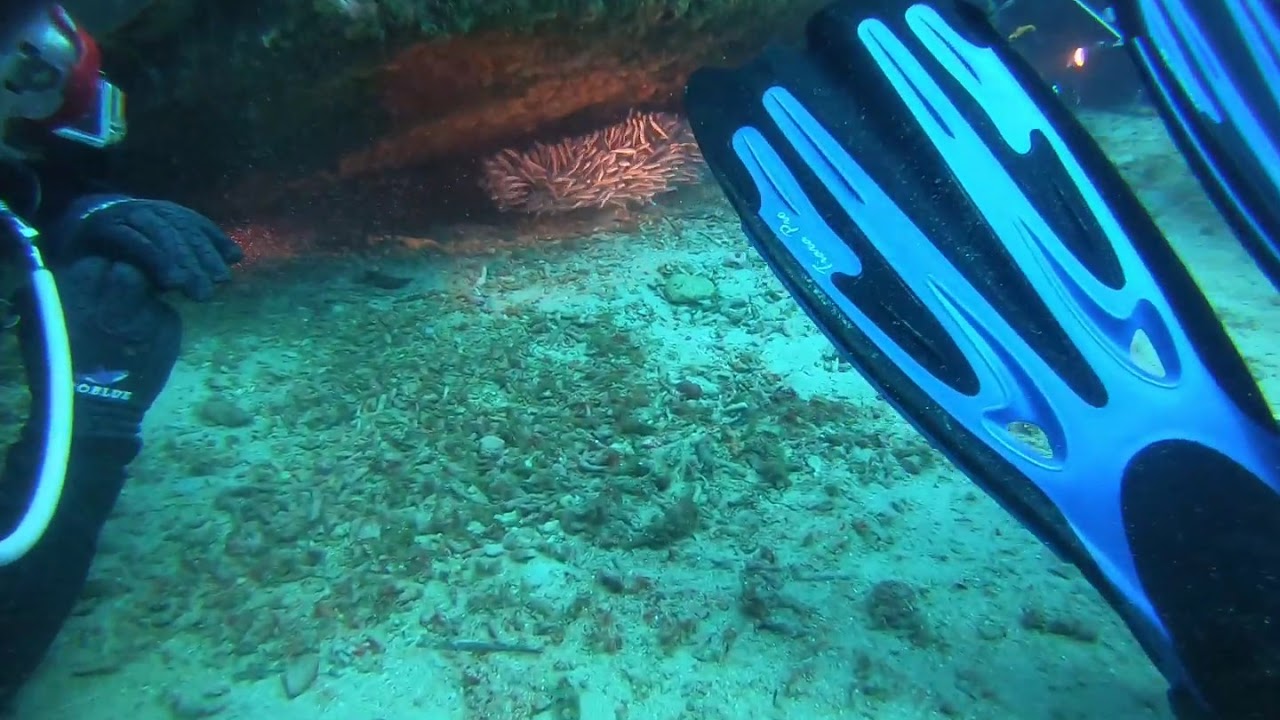This underwater photograph, taken from the perspective of a scuba diver, captures a vibrant, detailed scene near the ocean floor. The right half of the image prominently features the diver’s blue and black fins, adorned with white lettering on the left fin's top side. To the left, a second diver, clad in a black jumpsuit, black gloves with indistinguishable white wording, and red goggles, is visible. This diver is facing forward, with a white breathing tube emerging from their mouth. Below them stretches a white sandy seabed interspersed with brown vegetation. Towards the top of the image, a rock shelters a white sea anemone. In the upper right corner, another diver aims a light at the sea anemone, illuminating this underwater marvel. The entire scene is suffused with the turquoise hue of clear, underwater light.